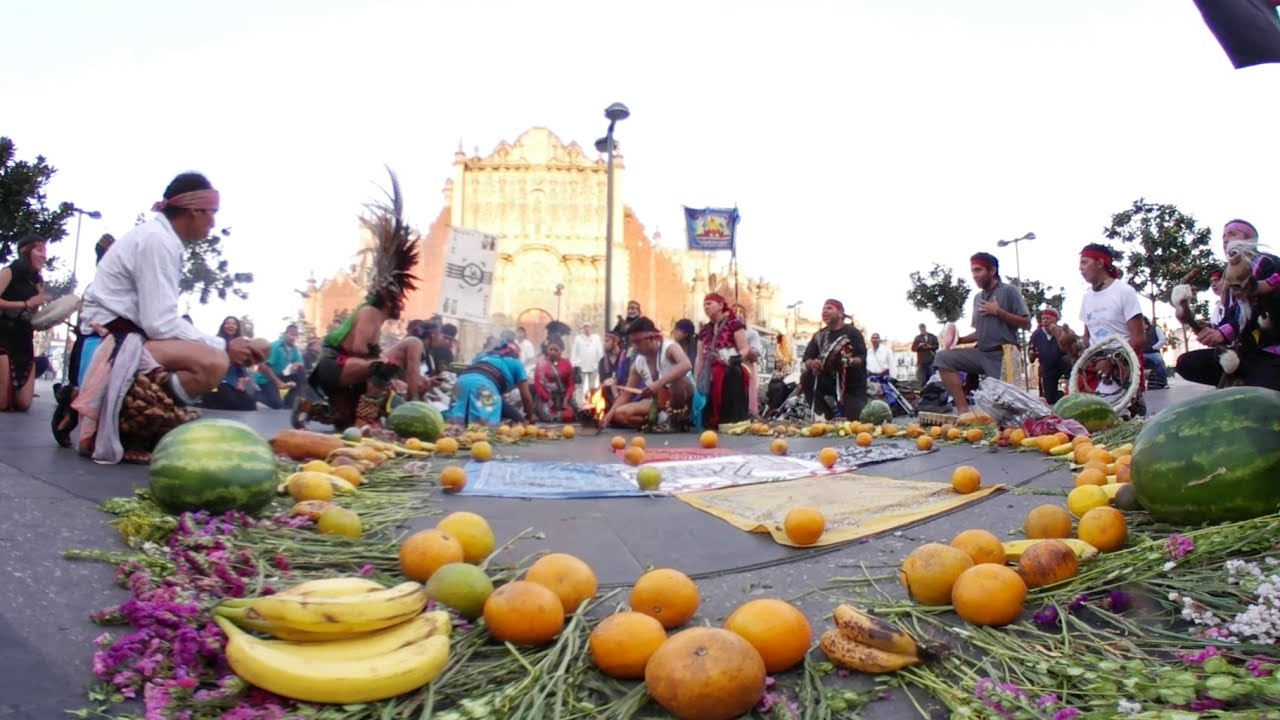In this outdoor scene, captured with a fisheye lens that curves the edges slightly upward, there is a gathering of people and an arrangement of fruits and objects on the ground of a paved area. The central focus features a circle of various fruits, including oranges, bananas, watermelons, and possibly mangoes. Intriguingly, some of the oranges are green, and there are also green stems with purple flowers and what appear to be asparagus stalks.

Surrounding this circle of fruits, a group of people with a slightly hippie appearance are either squatting or sitting. On the far left, a woman on her knees seems to be hitting a tambourine. Moving to the right, a man wearing a white shirt and a bandana with material around his ankles is kneeling. Another individual, notable for his feather headdress, appears to be squatting, and possibly participating in music-making with a tambourine. Additionally, the man on the far right seems to be holding maracas. Among these people, there's a person with flowers mounted on his head, his arm uncovered.

In front of these individuals, squares of cloth are anchored to the ground by some of the fruits. The background features a large, yellow and cream-colored building with an ornate arch top, possibly a church. Further back, a light post with dual lights stands behind the group. To the right of the building, a blue sign with an indecipherable emblem is visible. The sky above this scene is a solid white, adding a stark contrast to the colorful and lively foreground.